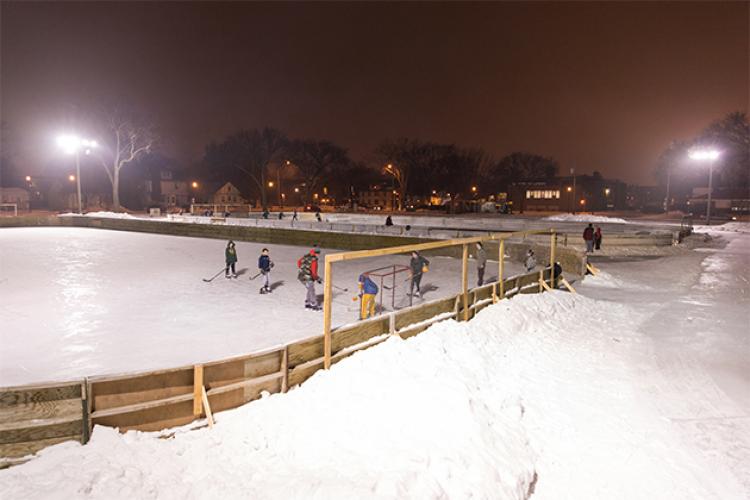This nighttime photograph captures a lively winter scene at an outdoor, makeshift ice skating rink, likely constructed by amateurs using various planks of wood. The rink is split into two sections: on one side, a group of six younger players—dressed in a mix of hooded sweatshirts, jackets, and a vest—engage in a spirited game of ice hockey. Among them, one player in yellow pants and a blue shirt appears to be tending the goal while another defends. On the other side, people are quietly skating. The rink is bordered by a snowy landscape with snow piled up along a fence and an adjacent icy street. The scene is illuminated by streetlights on both the left and right sides, casting a soft glow over the area. In the background, the vague outlines of trees and the twinkling lights from nearby houses and buildings in a residential neighborhood add depth and context to this wintery snapshot.